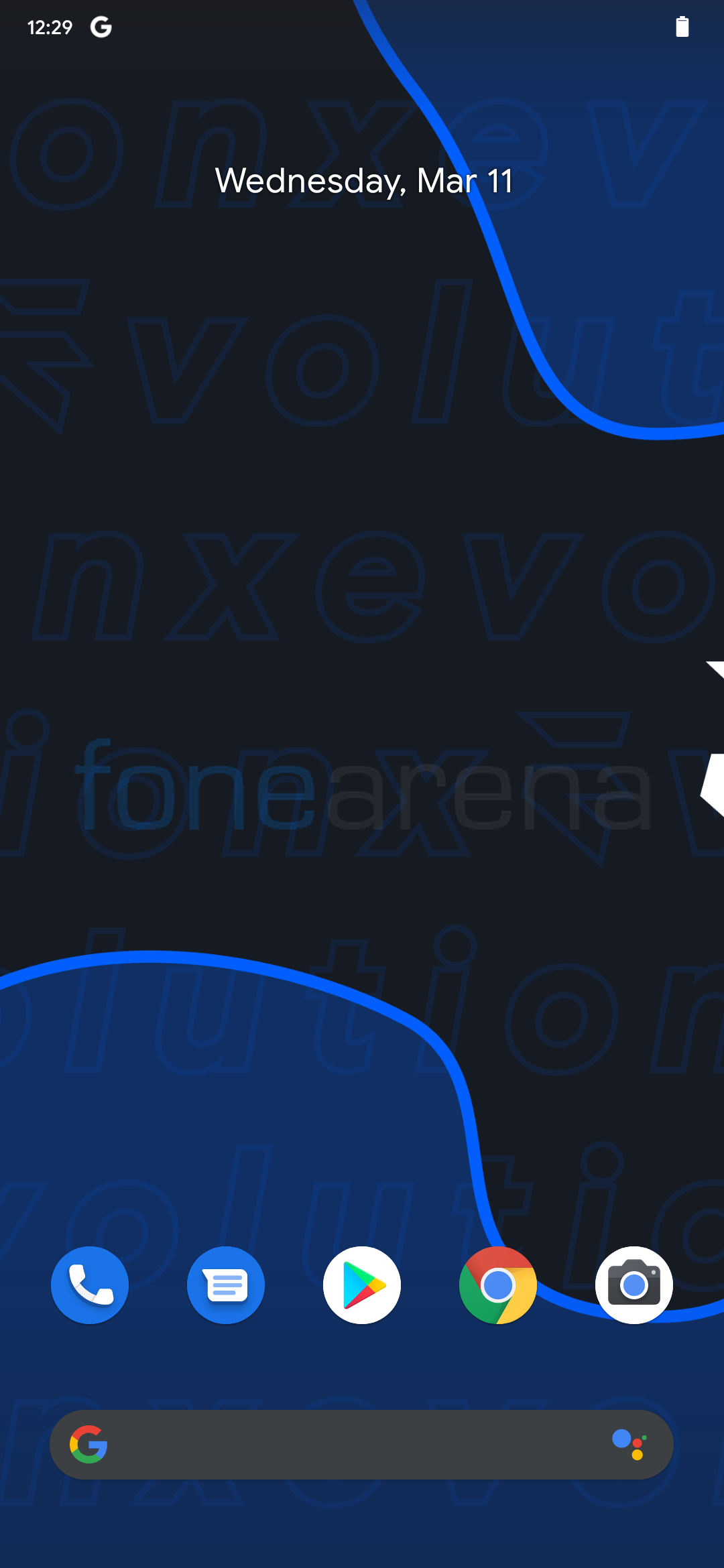The image is a screenshot of a smartphone display. The majority of the background is dark, primarily black, with various blue elements that create a contrasting layout. 

At the top right section of the screen, bordered by a light blue line that curves downward for about two inches before disappearing off the right edge, the background transitions into a darker blue shade.

On the left side near the top, the screen displays "12:29" in the top left corner, while a large "G" appears prominently on the right side. Adjacent to that is a small white battery icon. Centrally located and mostly set against the dark area with some overlap into the blue area is the text "Wednesday, March 11th."

Across the top part of the background, there is text that appears to say "ONXEV" followed by fragmented text "V O L U T," "N X E V O," and partial words that include "I O N X." These fragments appear to move off the screen to the right and are layered on top of each other, creating a chaotic yet structured look. Overlaid near the center, the word "F O N E" is depicted in blue text, next to an orange-ish area. Below this are fading letters "L U T I O N" and just beneath that, "O L U T I O N."

An inch from the bottom, within a blue border, various app icons are arranged. Starting from the left, these include a blue call icon with a white phone, a blue circle with a white text message icon, the Google Play icon, the Google Chrome icon, and a white circle containing a camera icon. Directly below these app icons is a black search bar. The search bar features the Google "G" on the left side followed by a small blue dot, a red dot, and a yellow dot on the right side.